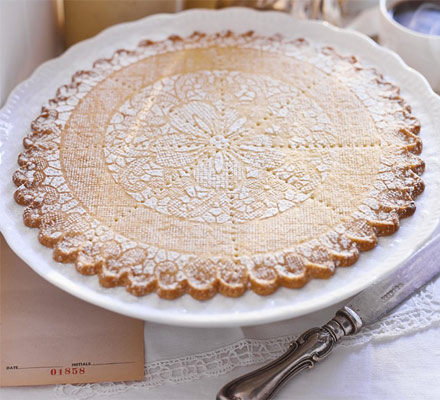In this photograph taken from a slightly angled overhead perspective, the focal point is an intricately designed pie crust resting on a white plate. The pie crust features ornate borders with carefully crafted floral designs. Concentric circles, each with a marbled pattern that connects with the floral elements, add to its elaborate appearance. A blank circle occupies the center of the crust, while dotted lines divide the pie into eight perforated slices, giving it a pre-cut appearance.

The surrounding setup includes a silver cutting knife with a semi-intricate handle placed beside the plate. The background is a white cloth, and a brown card or envelope partially peeks out from under the plate. A delicate layer of white powdered sugar lightly dusts the top of the pie crust, enhancing its visual appeal. The detailed craftsmanship of the dough along with the thoughtfully arranged setting makes this image a captivating display of pastry art.